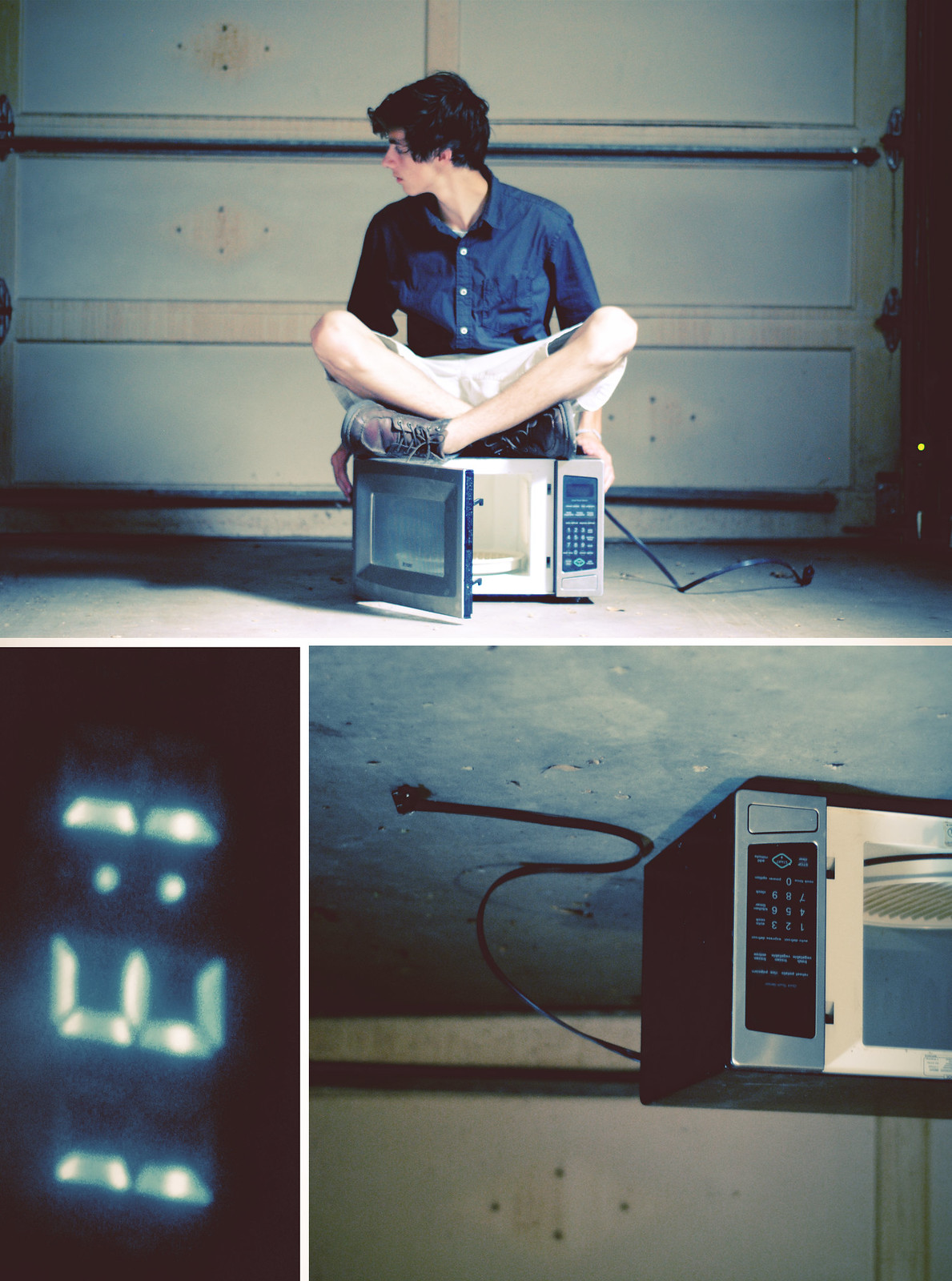The image is divided into three sections. The top section features a man with short curly hair and a light skin tone, dressed in a long-sleeved blue button-up shirt, white shorts, and black shoes with brown leather, sitting cross-legged on an unplugged microwave. He is looking to the left while holding the sides of the microwave, which has its door open, revealing a white interior and a little turntable. In the background, there is a white garage door. 

In the bottom left section, a close-up image shows the clock display of the microwave tilted 90 degrees to the north, showing "CED-131" in bright white text on a black background. 

The bottom right section features an upside-down view of the same microwave without the man. The microwave's black wire, originally extending to the right in the top image, appears on the left side and on the ceiling from this perspective.